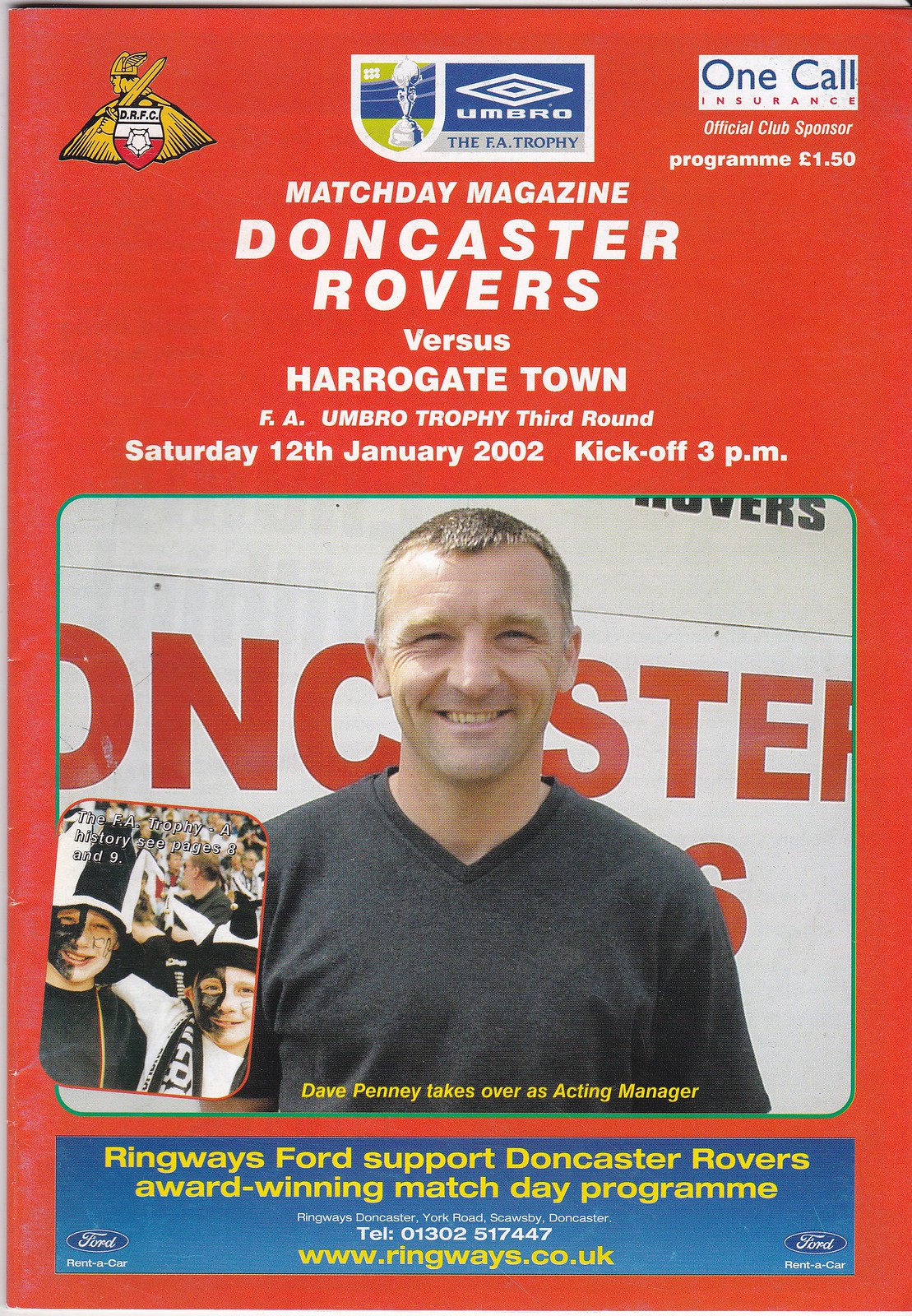This image is a scanned cover of a match day magazine program with a bold red background. At the top right, in a white box with blue text, it reads "One Call Insurance" followed by "Official Club Sponsor." Below this, in yellow, is the symbol for currency and "Program 1.50." The center prominently features an Umbro logo with the text "Match Day Magazine" underneath. It details the event: "Doncaster Rovers vs. Harrogate Town, FA Umbro Trophy, 3rd Round, Saturday, January 12, 2002, Kickoff 3 p.m." 

Beneath this text is a photograph of a white male, possibly a player or staff member, smiling and wearing a gray v-neck shirt. His short brown hair is slightly receding. A caption near him states, "Dave Penny takes over as acting manager." To his left, there's a small image of two children with faces painted, presumably in team colors. 

At the bottom, there's an advertisement for Ford, reading "Ringways Ford Support Doncaster Rovers Award-Winning Match Day Program." The ad includes a telephone number and a website in yellow and white text.